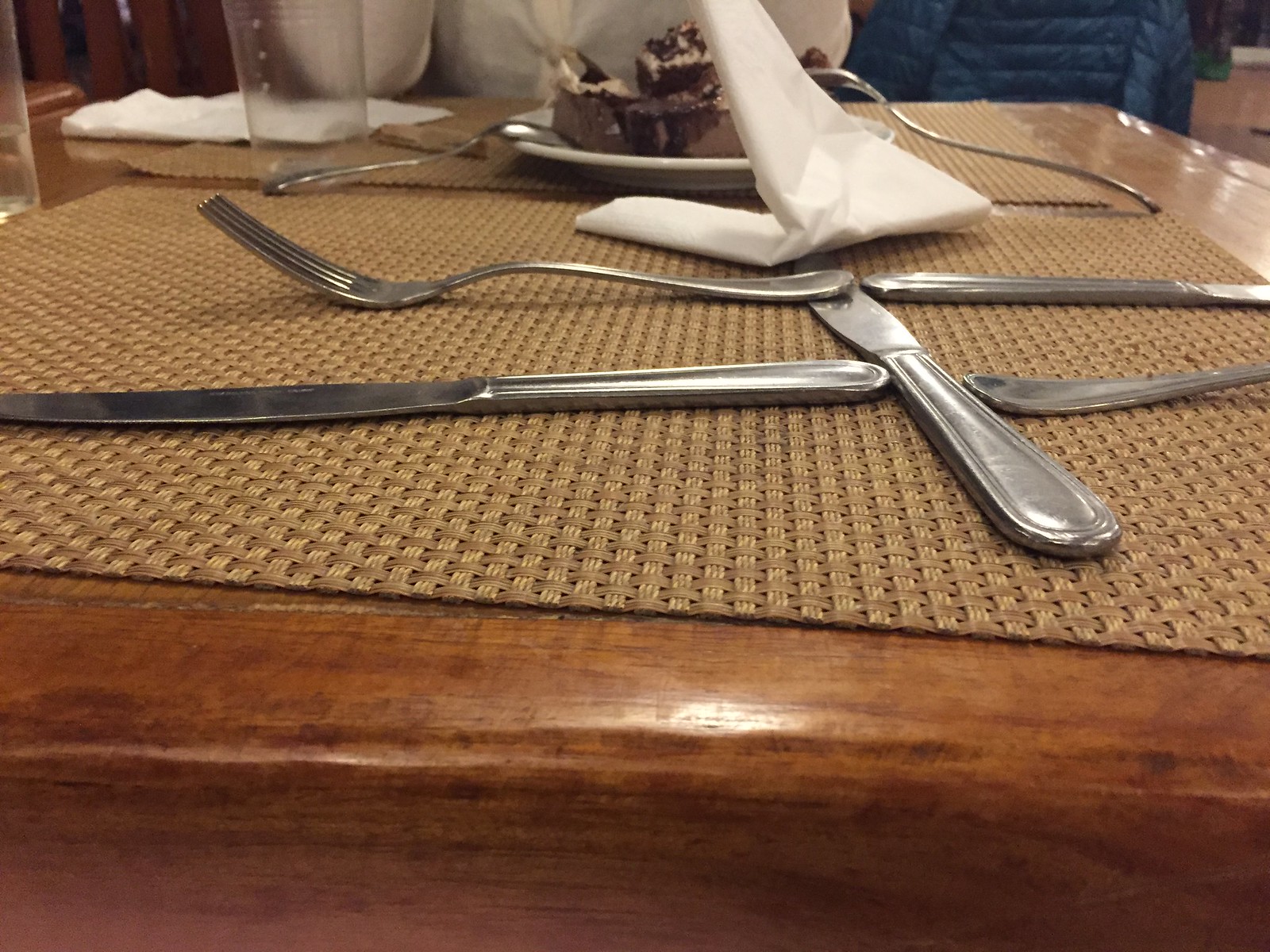This close-up photograph captures an intricately set dining table. The centerpiece features a tan, dark-tan basket weave mat bordered by brown wood. Silverware is meticulously arranged in a symmetrical pattern: on the left side, a fork is placed on top of a butter knife, while on the right side, the order is reversed with a butter knife above a fork; three butter knives are prominently noted. A plastic napkin lies beside empty restaurant-style hard plastic drinking cups. A delectable dessert, possibly a chocolate cake or sundae adorned with fudge, white cream, and chocolate flakes, sits on a small plate in the foreground. Utensils, including a spoon and a fork, rest upside down on the dessert. In the upper part of the image, a folded napkin is visible. A person in a white long-sleeved shirt, with their elbows resting on the table, occupies the background, alongside a hint of a blue jacket.